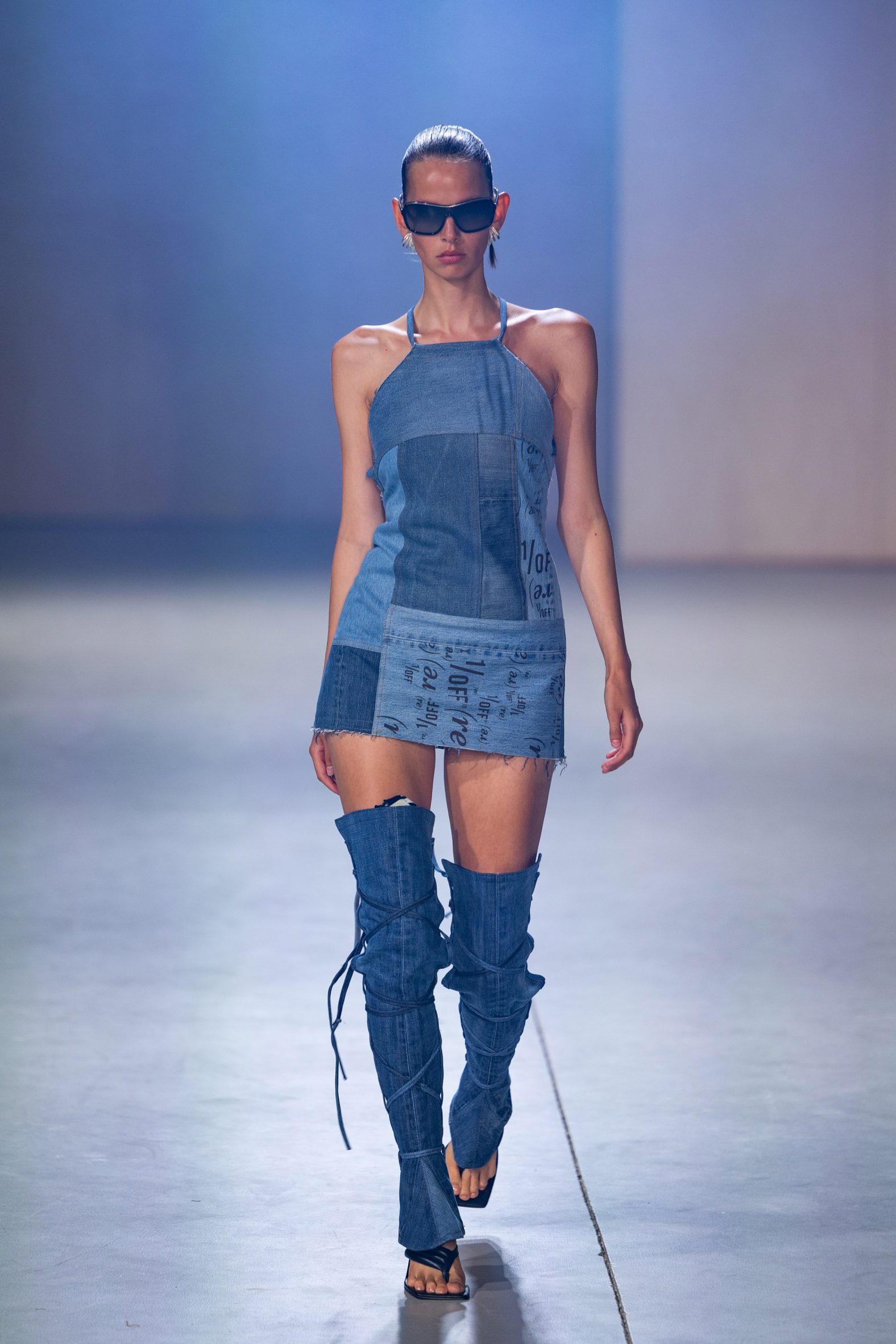A striking image captures an experienced female runway model confidently striding down the runway with a fierce, concentrated look. Her brunette hair is slicked back into a ponytail, and she sports dark, tinted sunglasses that add to her serious demeanor. Her outfit is a unique denim-on-denim ensemble: a blue denim dress made from various patches of jeans in different shades, from light to dark. The dress, resembling an apron, has a neck strap and is cut very short, barely covering her upper thighs. Engravings can be seen on the dress, adding a distinctive touch. On her legs, she wears thigh-high leg coverings made of dark blue denim with straps that wrap around. She pairs these with black, open-toed sandals that have a jeans-like appearance, creating a seamless denim look from her feet to her thighs. Accessorizing minimally, she dons a single long earring on her left ear, reinforcing her poised and experienced runway presence.